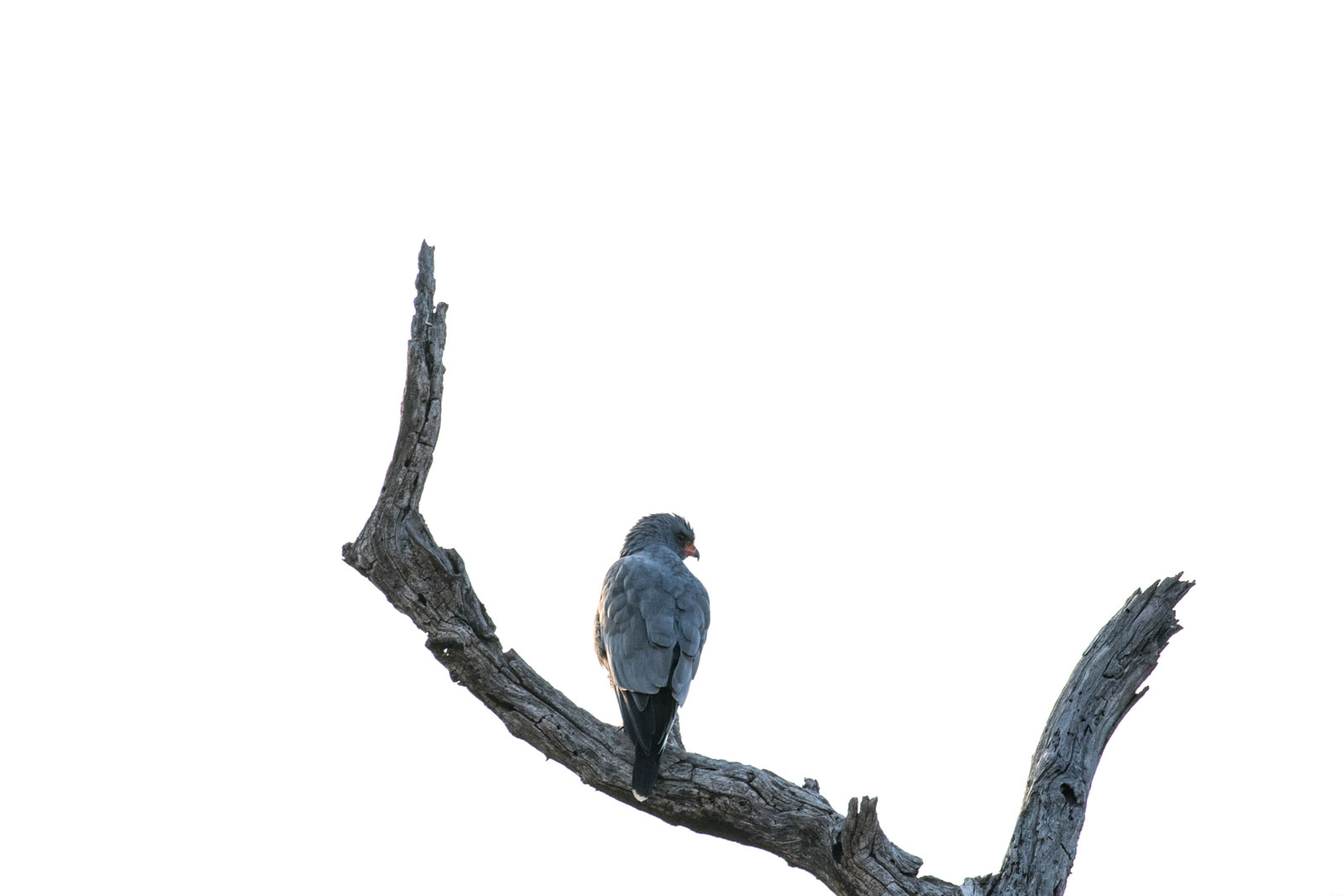The landscape-oriented color photograph captures a small, blue-gray bird perched centrally on a gnarled, weathered tree branch that forks in a distinctive V shape. The background has been photographically removed, resulting in a stark white backdrop that accentuates the detailed realism of the scene. The tree branch, emerging from the bottom right, has one longer, slightly upward-curving arm to the left and a shorter, broken-off arm to the right. The bird, identified as a gray falcon or owl with soft, fluffy feathers, has its wings folded neatly against its body. It sports a sharply curved yellow-orange beak and small black eyes, with its head turned right, peering back over its shoulder. Its straight tail feathers are primarily black, with a touch of white at the tips. The scene evokes a sense of stillness and introspection, with the bird perched serenely on the bare, possibly dead tree, surveying its surroundings.